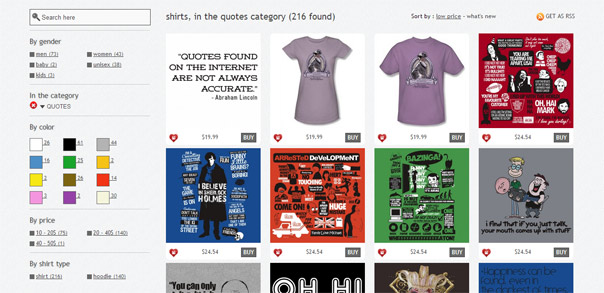The image appears to depict a webpage from an unidentified website dedicated to selling shirts. In the upper left-hand corner, there is a search bar labeled "Search here." Below the search bar, a category titled "Shirts" is listed, and within the "Quotes" subcategory, a total of 216 items have been found. Users have various sorting options, including sorting by low price, newest items, or as RGS. Additionally, there are filters to sort by gender, color, and price, with color swatches displaying a variety of hues.

The merchandise includes a wide range of shirt types and hoodies, characterized by busy graphic designs and quotes. One notable shirt displays the phrase, "Quotes found on the internet, not always accurate.” The shirts come in multiple colors, such as purple, blue, red, green, and pink. The graphics on the shirts are vibrant and varied, including cartoon characters and other eclectic designs. One gray shirt features four partially visible designs, one of which has the text "Oh, hi" with the bottom portions cut off. The overall layout showcases a vibrant and diverse collection of shirts for different preferences.